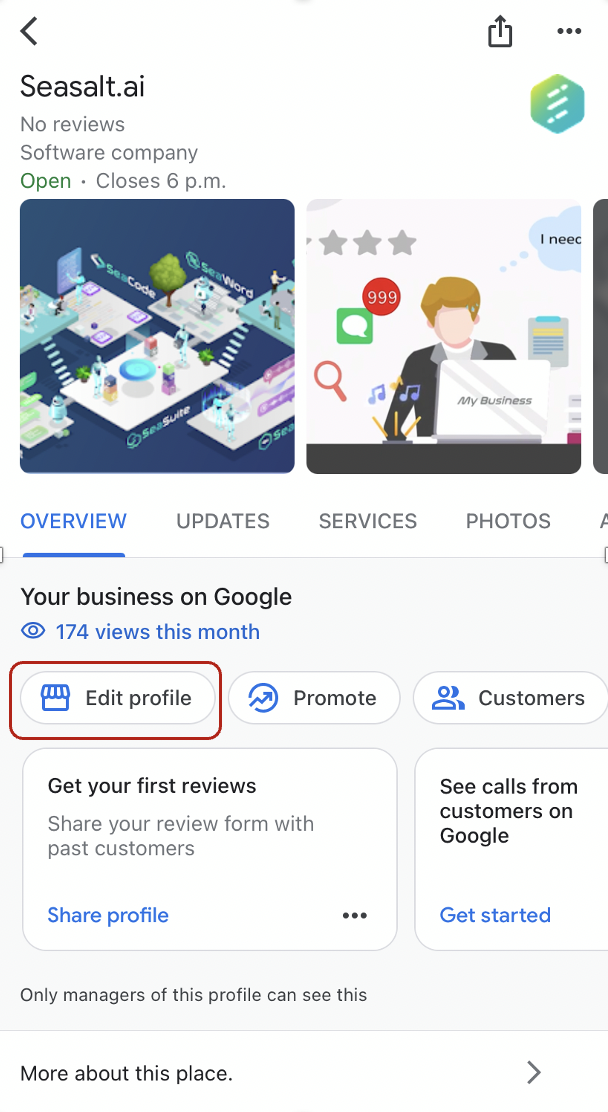At the top of the web page, the text "CSALT.AI" is prominently displayed in black letters. Directly beneath it, in smaller black text, it reads "No Reviews Software Company" and provides the business hours, "Open Closed 6pm."

Below this header are two square images. The first image is an aerial view of various small, interconnected squares. One square features a tree, another depicts a table with three small figures (resembling stick people or bobble people) gathered around it, and there are small staircases connecting these squares, some of which are floating while others rest on the ground.

The second image contains three gray stars, a red circle, a green square with a speech bubble, a red search button, musical notes, and a character with red hair dressed in a black suit and white shirt, working on a laptop.

Further down the page, the categories "Overview," "Updates," "Service," and "Photos" are listed, with "Overview" highlighted in blue and the others in black, spanning from left to right. Following this section is a statement indicating that the business has received 174 views this month on Google. Buttons labeled "Edit profile," "Promote," and "Customers" are aligned from left to right.

The call-to-action section encourages users to get their first reviews by sharing a review form with past customers and sharing the profile. Next to this section, a rectangle prompts users to "See calls from customers on Google" with a "Get started" button.

At the bottom of the page, it states in black letters that "Only managers of this profile can see this," followed by more information about the place and an arrow button pointing to the right.